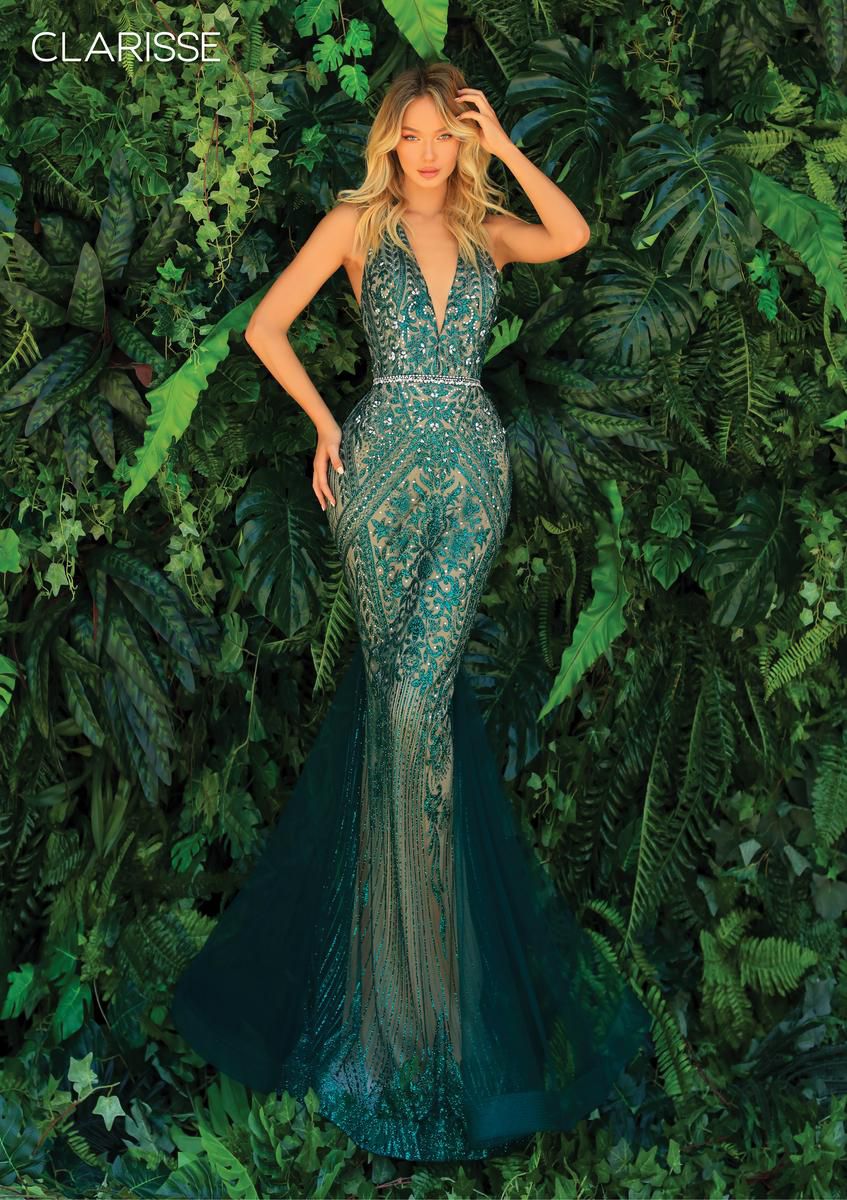This is a highly stylized magazine advertisement featuring a tall, blonde Caucasian model positioned against a lush, verdant green backdrop filled with tropical foliage and ferns. The setting appears to be a dense jungle or forest with an abundance of greenery. The model stands centrally, wearing a luxurious, sparkly teal green strapless gown that contrasts slightly with the darker green vegetation behind her. The dress features a deep plunging v-neckline, tying behind her neck, and a form-fitting bodice that flares out into a mermaid-style skirt at her knees. Her right arm is bent at the elbow with her hand resting on her hip in a classic teacup pose, while her left arm is extended outward at shoulder height, with her hand lightly threading through her long blonde hair. In the upper left corner of the image, the word “CLARISSE” is prominently displayed in bold white capital letters. The entire scene exudes an impression of elegance and natural beauty.